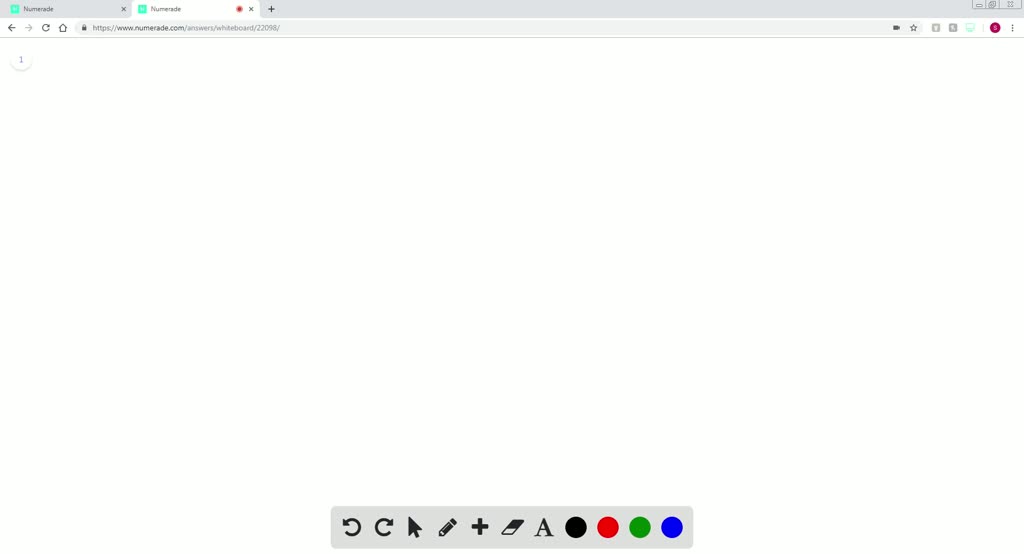The image displays a computer screen with two open browser tabs. The current tab's logo is a mint greenish-blue color. A small red circle, indicating active listening or recording, is visible. The webpage in this tab is primarily white. Although no mouse cursor is visible, the bottom section of the screen features a toolbar with various color options including black, red, green, and blue.

The toolbar contains several icons: a "little a" for text input, an eraser, a plus button, a pencil, and an arrow. Additionally, there are back and forward navigation buttons, implying this could be a drawing or annotation tool.

In the top right corner, positioned under the standard browser back, forward, and refresh buttons, there is an icon resembling a small circle with an "i" inside it, indicating information or help. On the opposite side, typical window control buttons for minimizing and closing the tab are present.